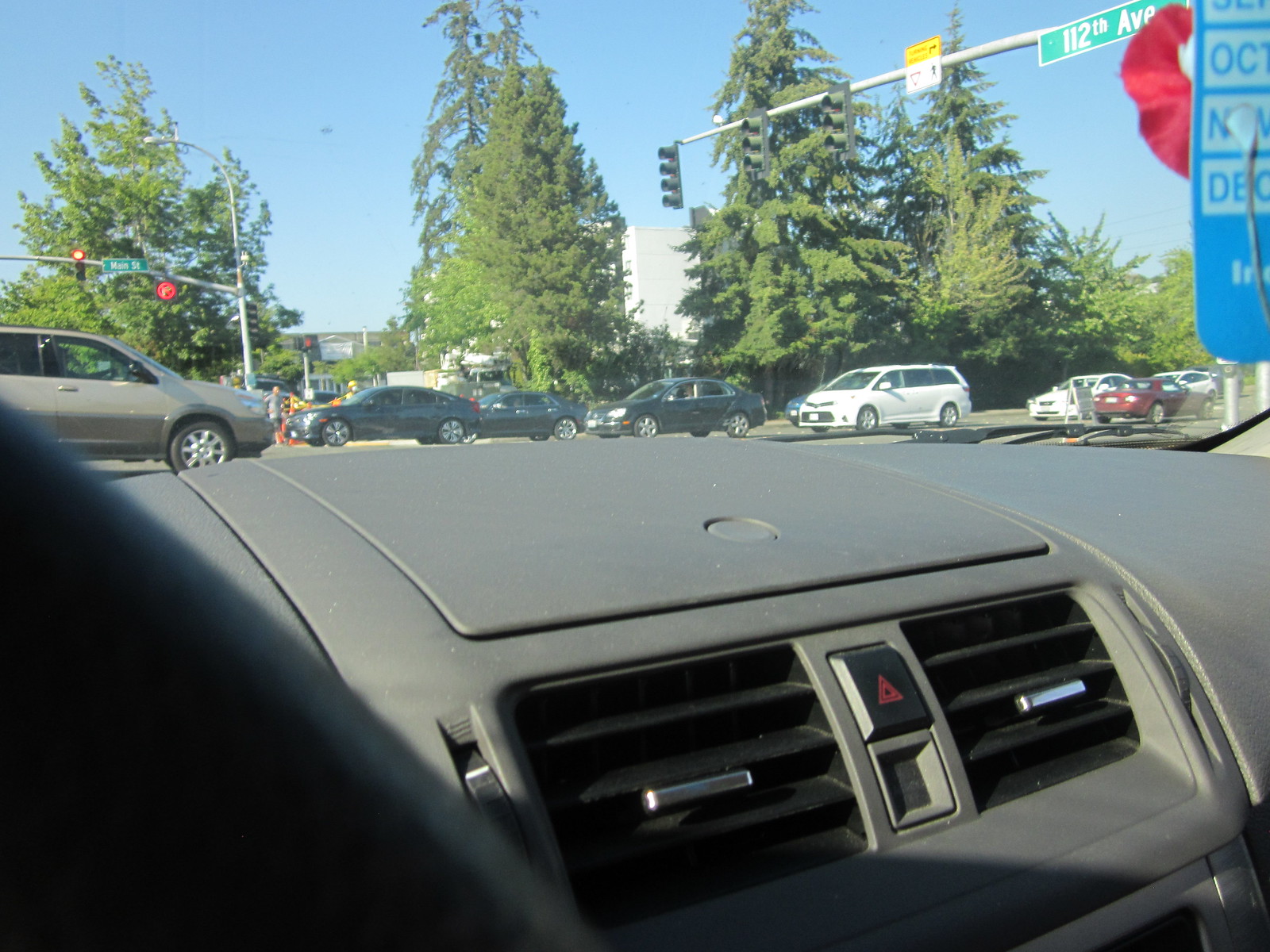The image showcases the interior of a vehicle, focusing prominently on the gray plastic dashboard. Central to the dashboard are air vents, which feature a silver handle and a red triangle button, indicative of the hazard lights. Above the dashboard, the scene extends to an exterior view, where a clear blue sky frames a row of pine trees. On the right side of the image, a blue road sign is visible, displaying text related to Iron Toad's Avenue. Additionally, a white sign with a yellow dot is present, possibly for traffic direction or caution. The traffic light is illuminated red, signaling a stop, and various cars in colors like white, gray, black, and red are seen waiting at the intersection.